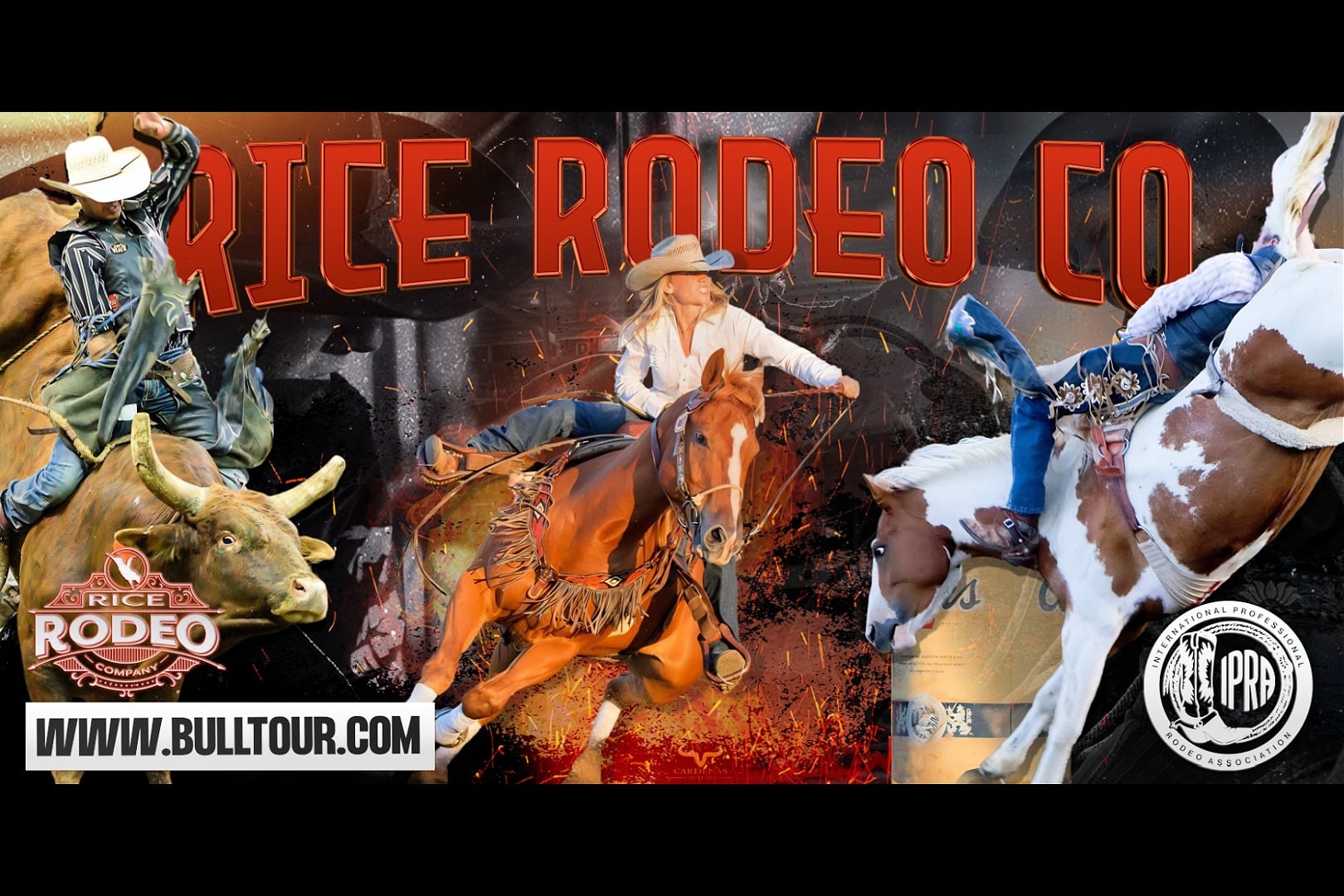The poster for the Rice Rodeo Co. features a striking, glossy, rectangular design with a dark black background. Dominating the top in large, bold red capital letters is "RICE RODEO CO." Centrally placed, a blonde female rider in a white button-down shirt, jeans, and a cowboy hat is astride a brown horse in mid-gallop. To her left, a man in a white cowboy hat, blue button-down shirt, and jeans is fiercely riding a brown bull. On the right, a spirited brown-and-white horse is captured mid-leap with a rider clinging on. In the bottom left corner, the URL www.bulltor.com is clearly displayed, while the logo for the International Professional Rodeo Association (IPRA) adorns the bottom right. The overall clarity and natural lighting of the image enhance its vibrant and energetic depiction of rodeo action.